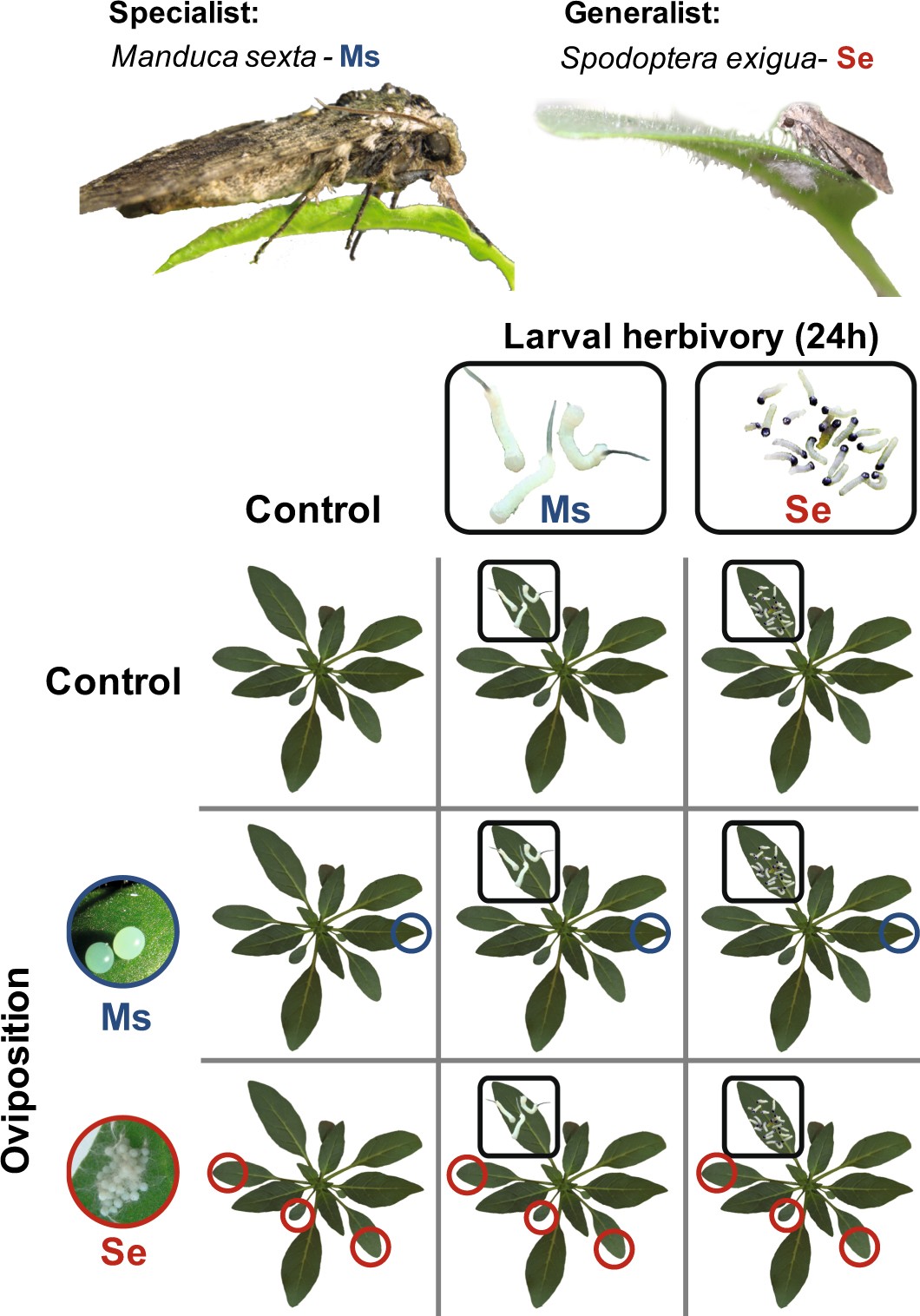The image is a detailed diagram illustrating the interaction of insects with leaves, focusing on two types of insects and their impact over a 24-hour period. At the top, there are two images side by side: the left image is captioned "Specialist Manduca sexta-MS" showing a large, brown locust-like insect on a green leaf, while the right image is captioned "Generalist Spodoptera exigua-SE" depicting a smaller, greyish insect on a fuzzy green leaf. Below these images is the text "larval herbivory 24H," accompanied by two small squares labeled "MS" and "SE." Under this section is a 3x3 grid of nine images that display various leaves with bite marks and migration traces made by the insects. The first column is labeled "Control," while the second and third columns are labeled "MS" and "SE" respectively, showing the comparative impact of the two insect types on the leaves.